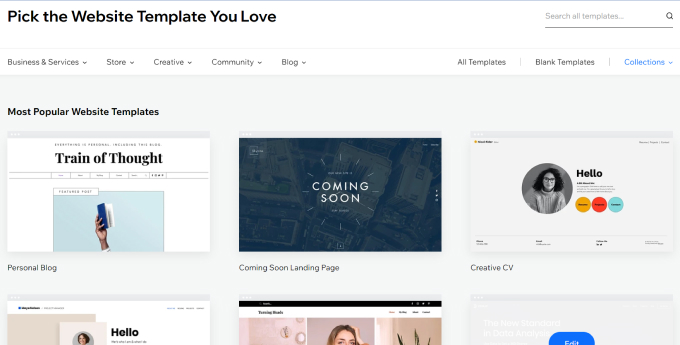In this image, we observe a website page dedicated to selecting website templates. The design predominantly features a clean white background accented with gray and black text. At the top of the page, a prominent heading reads "Pick the website template you love," with a search box to the right labeled "Search all templates…" accompanied by a magnifying glass icon.

Directly below this, there is a navigation bar with several sections, where the "Collections" section is highlighted in blue. To the left of "Collections," we can see the "Blank Templates" and "All Templates" sections.

On the left-hand side of the page, there is a menu offering additional categories such as "Business and Services," "Store," "Creative," "Community," and "Blog."

Within the "Collections" section, the page showcases the "Most Popular Website Templates." Among these, we can identify the following templates:
- **Personal Blog:** This template features text reading "Train of Thought" and an image of a hand holding a book.
- **Coming Soon Landing Page:** Displayed with a central "Coming Soon" logo.
- **Creative CV:** This template includes an icon of a woman with a "Hello" next to her name, surrounded by various bubbles.

There are three other template images partially visible below these. One features a blue "Edit" button, another shows a woman with her hand on her head along with a "Hello" icon, and the last one includes a woman’s picture.